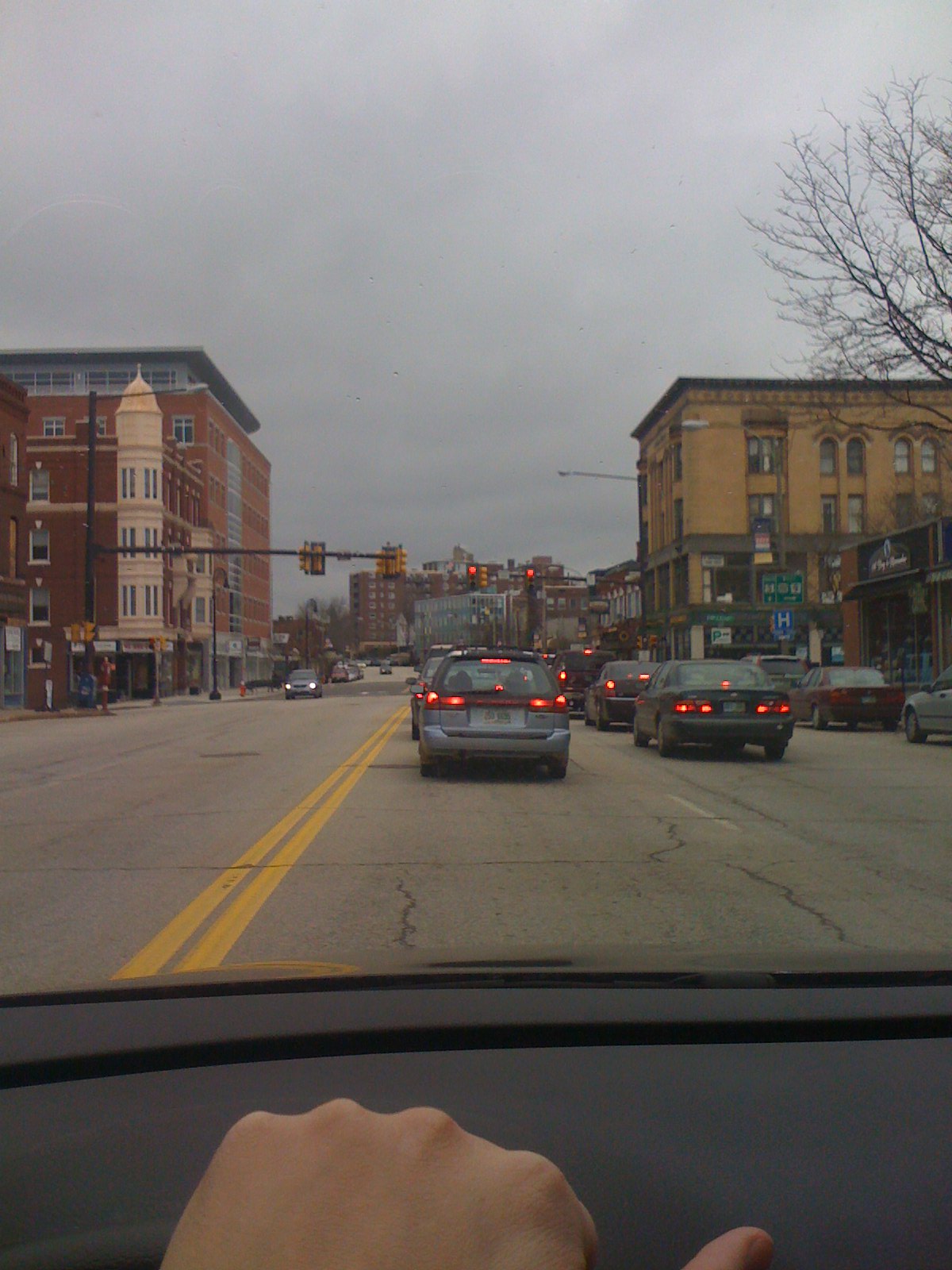The image presents a detailed view from inside a vehicle stopped in traffic. This vertical-oriented photograph captures the scene looking through the windshield. In the foreground, the top of the dashboard is visible, with the driver’s left hand resting on top of the steering wheel. Oddly, this hand appears somewhat computer-generated and lacks realistic detail. The thumb is positioned on the right side, angled slightly clockwise.

Beyond the dashboard, the urban street comes into view, illuminated by the red brake lights of the cars directly ahead, indicating a halt at a traffic light. The clear yellow dividing line on the road distinguishes the lanes. On the left side, cars heading in the opposite direction are also paused at the traffic light.

In the distance, the urban setting features structures that resemble downtown buildings, approximately four stories tall, positioned beyond the traffic light. Directly ahead and further away, various buildings, including an apartment complex, add to the cityscape, contributing to the bustling yet momentarily still atmosphere of the scene.